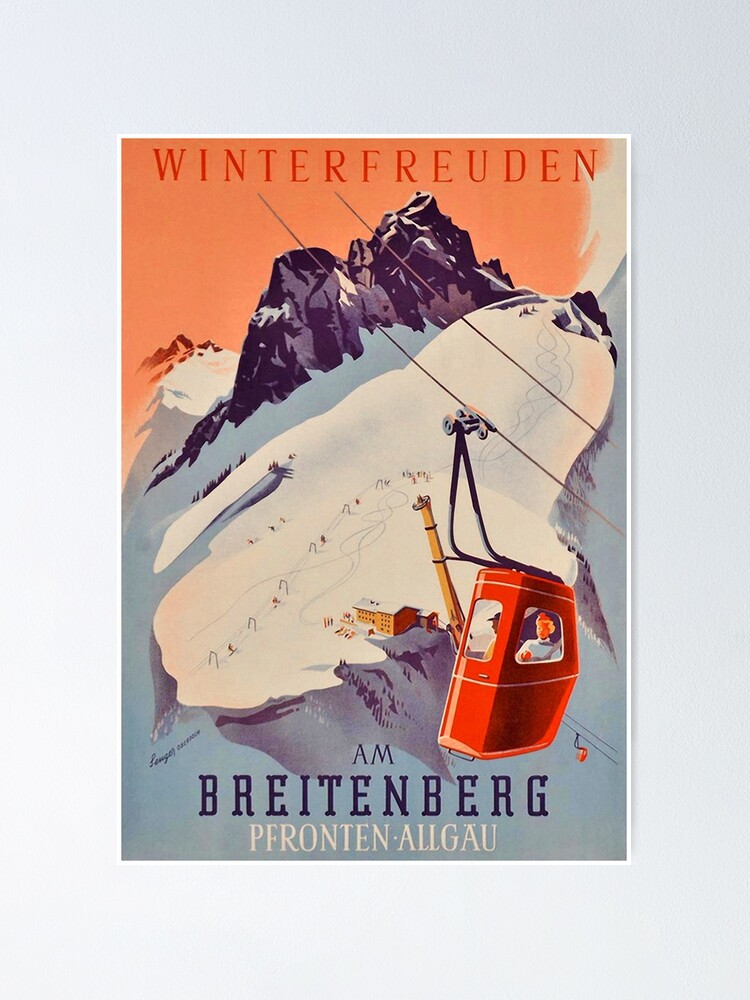This is an image within a white picture frame, possibly sized at 11x14 or 8x10 inches. The artwork depicts a whimsical snow-covered scene featuring a red car suspended midair by cables. Inside the car, a man and a woman can be seen. The backdrop consists of a purple-hued mountain and a blanket of snow. The image includes the text "W-I-N-T-E-R-F-R-E-U-D-E-N" at the top. At the bottom, it reads "A. M. B-R-E-I-T-E-N-B-E-R-G," and just below that, it spells out "P-F-R-O-N-T-E-N A-L-L-G-A-U."